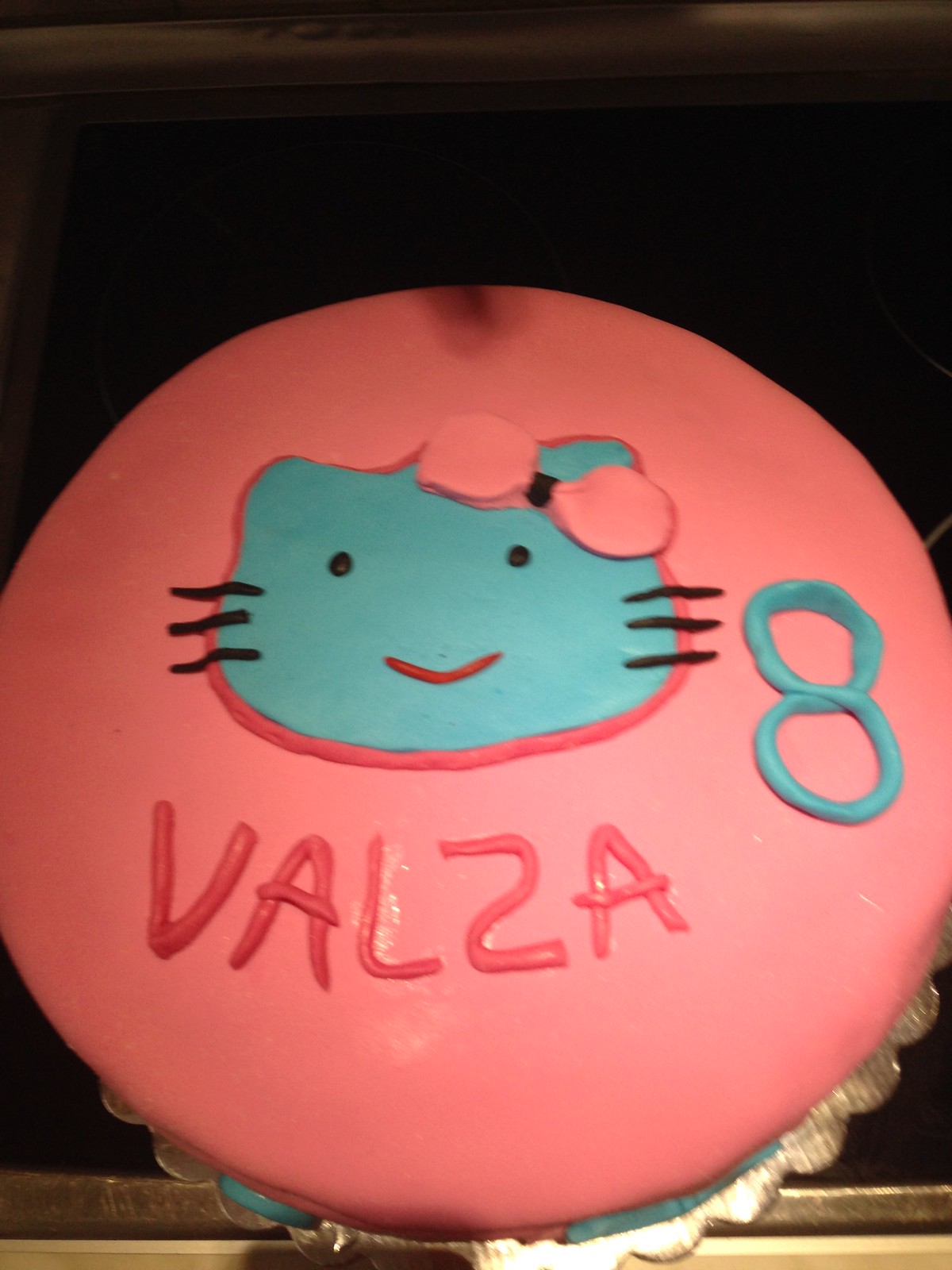This is a photograph of a round, pink fondant-covered cake, clearly designed to celebrate Valza's 8th birthday. The centerpiece of the cake is a charming depiction of a cartoon cat, reminiscent of Hello Kitty, featuring an aqua green face, simple black dot eyes, a red smiling mouth, and three black whiskers on each side. The cat is adorned with a large pink bow on the upper right corner of its head. The name "Valza" is written in red icing across the cake, matching the aqua green numeral "8" that indicates Valza's age. The cake appears to rest on a metallic tray or gold doily and is positioned centrally in the photograph, which has a dark background. The image is slightly blurry, suggesting it was taken casually, yet captures all the fond details of the cake's decorative elements.